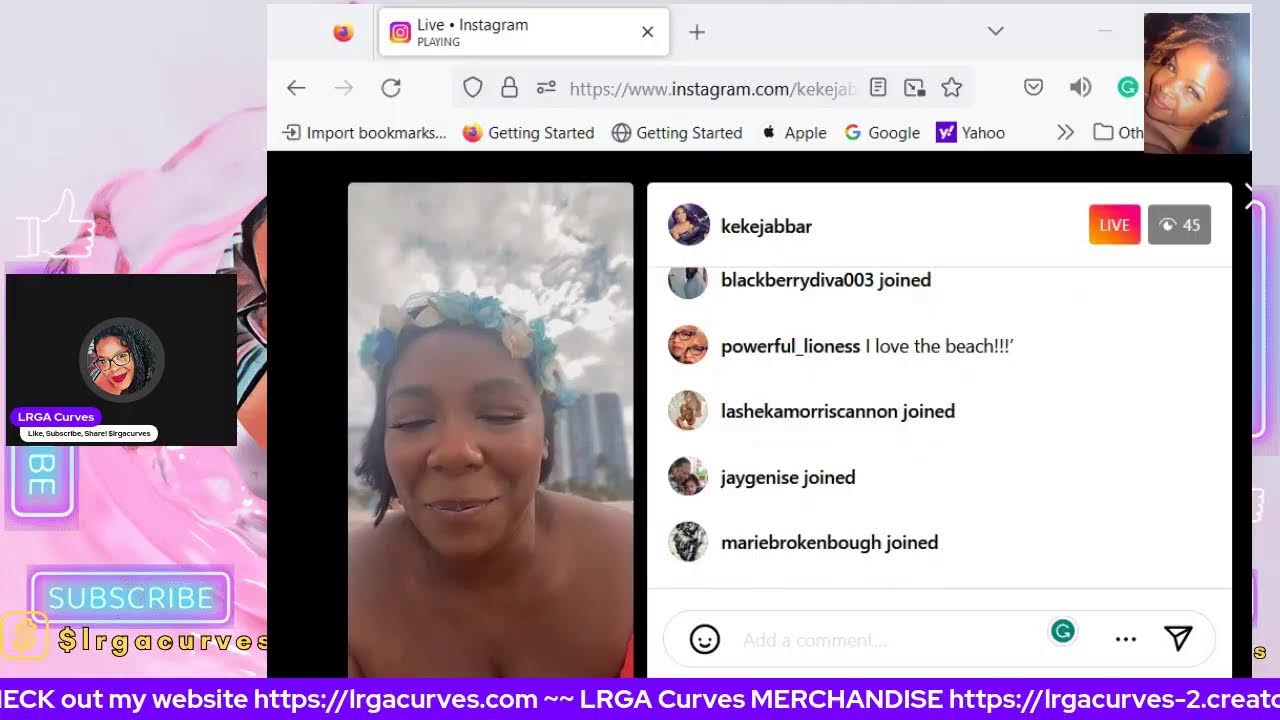Screenshot of a Firefox browser window displaying an Instagram live video. The tab at the top is titled "Live Instagram Playing," indicating that the video is streaming live. On the left side of the screen is a live video of a young Black woman with her eyes closed and smiling blissfully at the camera. She is adorned with a crown of flowers or a flowery hat and is wearing a brightly colored, low-cut dress or top, possibly in shades of pink or orange. Due to the close-up, her attire is not fully visible, but her radiant expression stands out.

On the right side of the screen, there's a list of user handles of the 45 people currently tuned into her live stream. Some notable handles include "kekejabbar" and "blackberrydiva003." A user with the handle "Powerful_lioness" commented, "I love the beach." Various other participants are also listed as having joined the live session.

In the background, the browser window appears to reveal the desktop of the person streaming the live video or someone associated with her. The desktop is adorned with promotional content such as "Subscribe," "Like," and "Check out my website: https://lrgacurves.com" providing additional engagement avenues for viewers.